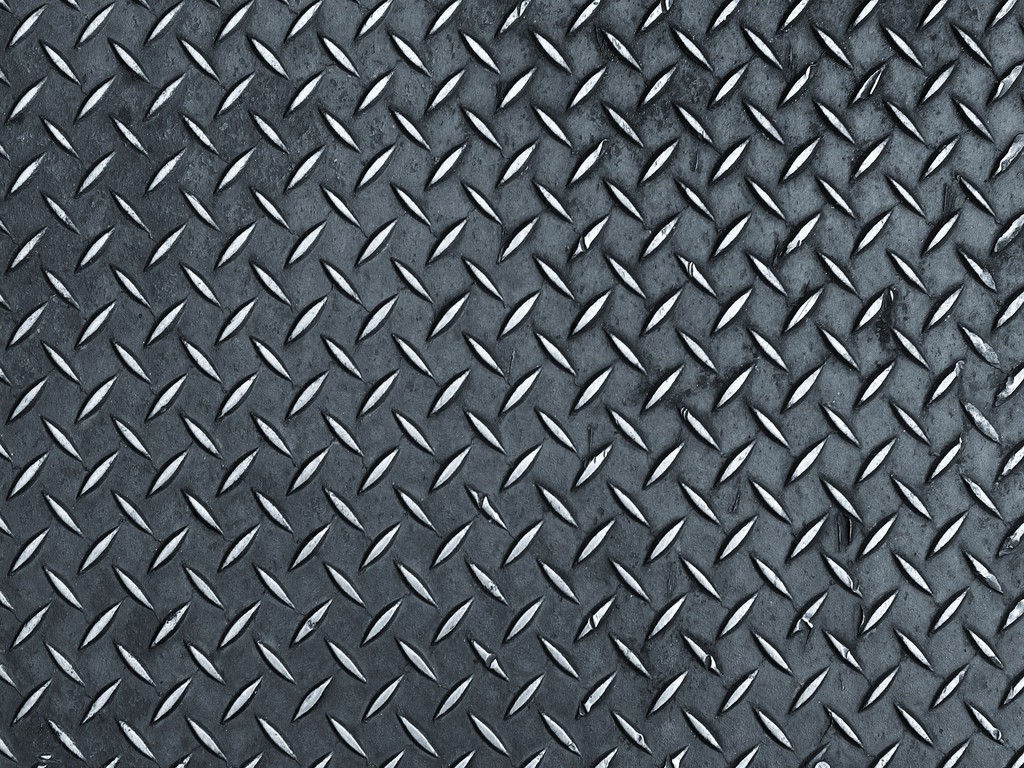The image features a close-up of a gray, textured metal sheet with an alternating pattern of elongated diamond-shaped protrusions, also known as a diamond plate. The protrusions are a silvery white color and are designed to prevent slipping, a common characteristic of surfaces used in industrial settings or on fire escapes. The pattern alternates direction with each row: the first row's diamonds slant from bottom left to top right, the second row from top left to bottom right, and this alternating sequence continues throughout the entire sheet. When observed from a distance, the alternating pattern creates an illusion of forming small squares. The entire image focuses solely on this metal texture, filling the frame completely.